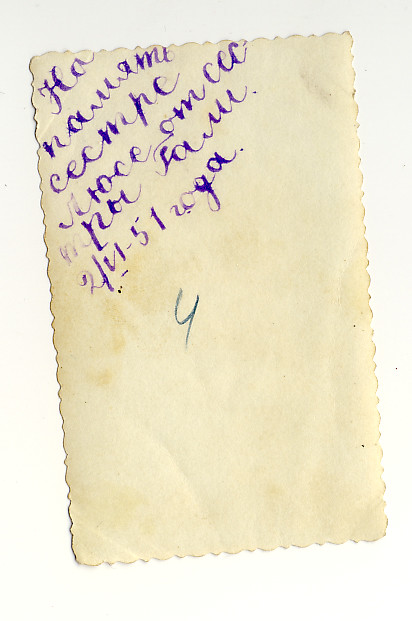An angled view reveals a vintage photograph with scalloped edges, lending it a classic aesthetic. The aged paper has taken on a yellowish hue, accentuated by noticeable yellow marks towards the center left. The photograph's reverse side features a handwritten note in a foreign language, penned in thick blue marker, descending from the top left corner. In striking contrast, the number "4" is prominently inscribed in blue ink at the center of the photograph, standing out against the white background. The combination of aged paper, scalloped edges, and varied ink styles adds a depth of historical intrigue to this captivating image.